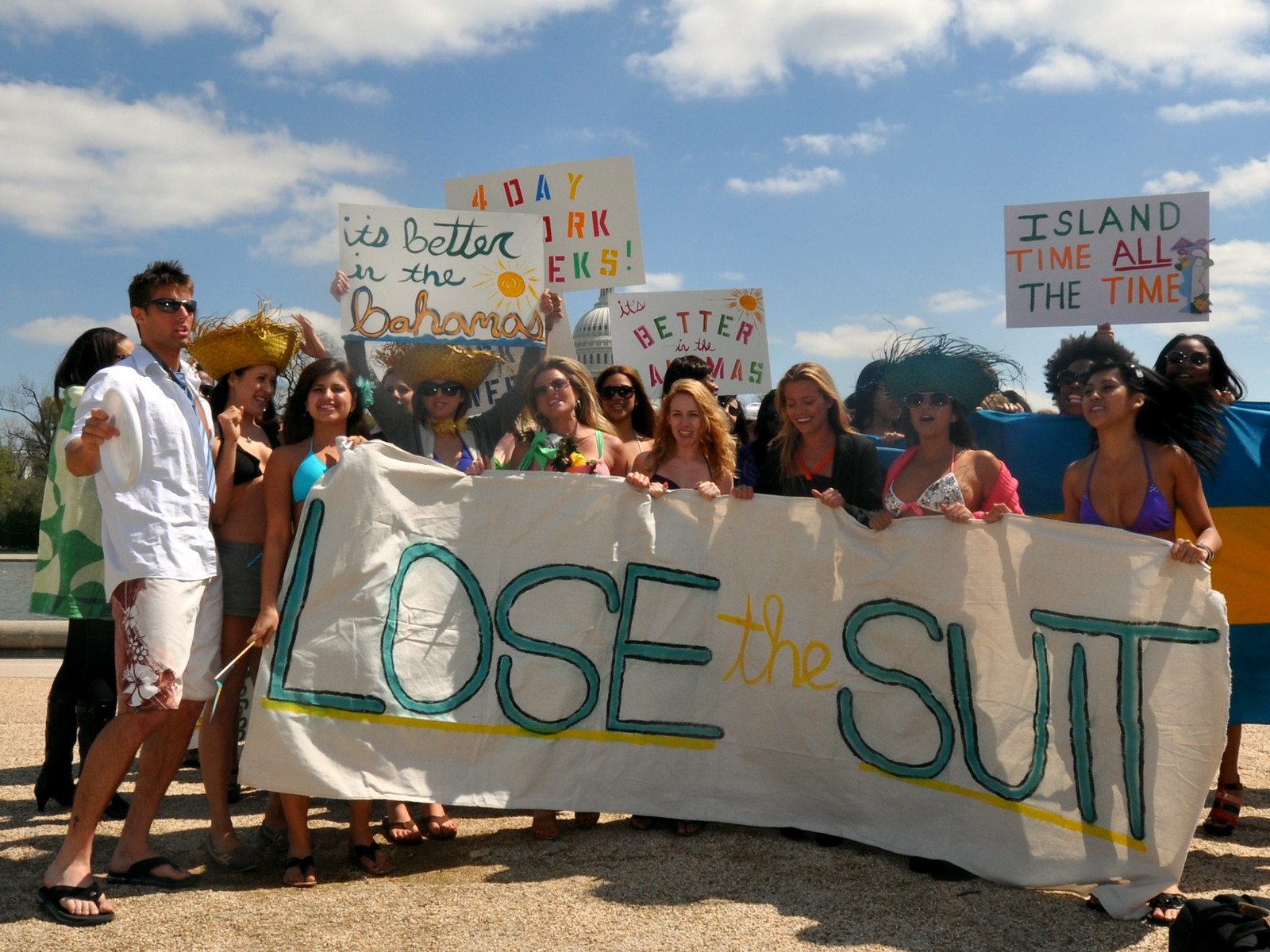The image captures an outdoor demonstration on a sunny day, likely in a tropical location such as the Bahamas, given the signs and attire. Central to the image is a group of college-aged individuals, around 20-22 years old, holding up a large homemade banner on a sheet or fabric. The banner prominently features the phrase "Lose the Suit" in green and yellow letters, underlined in yellow. On the right side of the group, a participant holds a sign reading "Island Time All the Time," while on the left, there are three sequential signs stating "It's Better in the Bahamas," "Four-Day Work Week," and "Better in the Bahamas Again." The participants are dressed for warm weather, wearing shorts, bathing suit tops, and sandals. Among them, a man stands slightly apart from the banner to the left, wearing a white short-sleeve button-up shirt, white swim trunks with a floral pattern, black sandals, and sunglasses. The sandy surface on which they stand and the light blue sky with some clouds above contribute to the tropical and summery atmosphere of the scene.